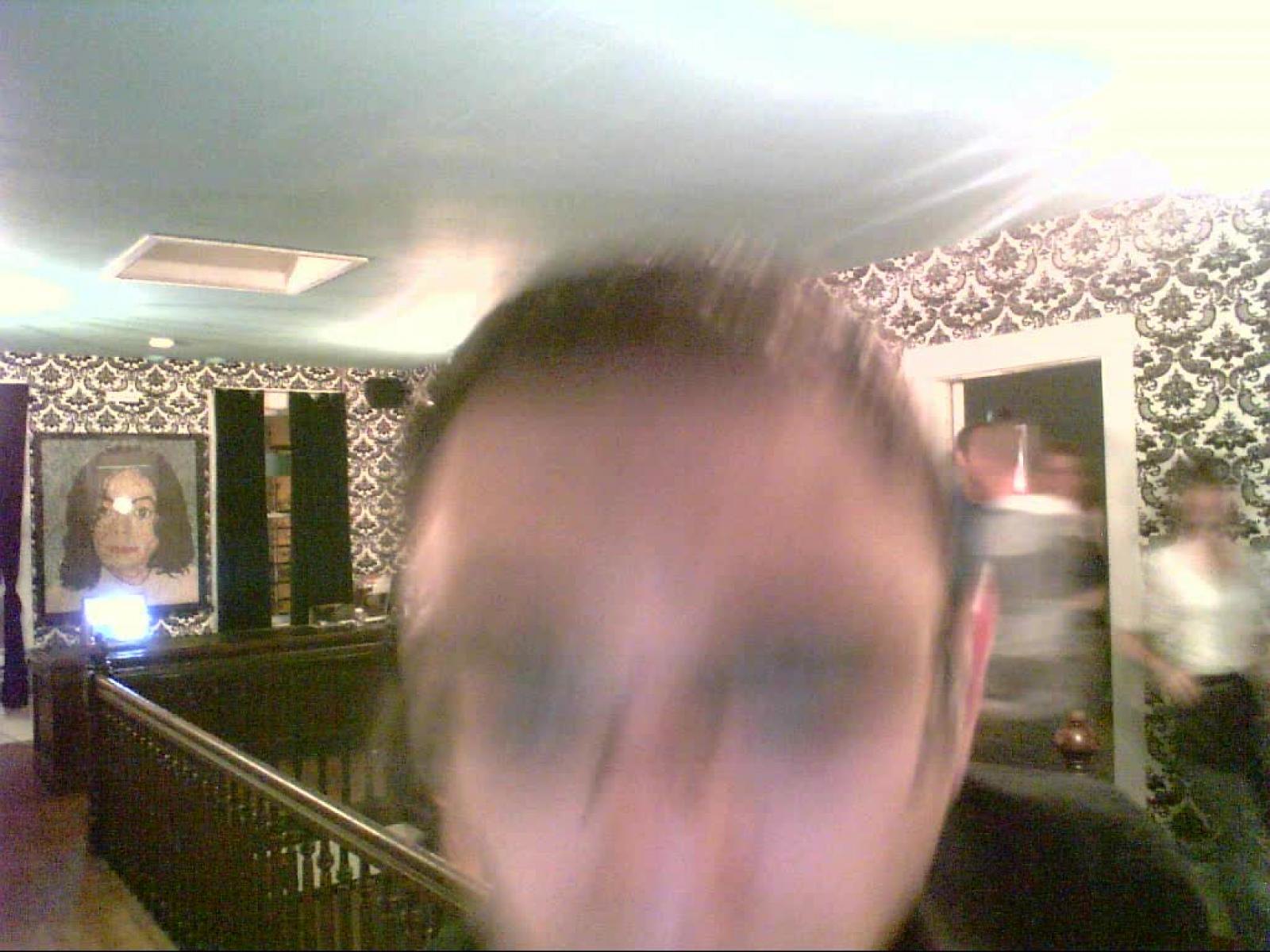The ceiling in the image is predominantly white, accented by lighting fixtures on the top right and left, as well as on the left side. At the background, there's a notable image or painting of Michael Jackson, adding a sense of charisma to the scene. The walls are adorned with white wallpaper featuring a unique black ribbon pattern, interspersed with circular designs that showcase images of bicycles. In the bottom right corner, a group of people is emerging from a doorway, but they appear blurred. Among them, one person in a blue shirt and another in a white shirt with black pants are somewhat distinguishable. The foremost individual, with short hair and glasses, is very close to the camera, although their features are also blurred. Adjacent to these people, wooden handrails are visible, leading towards a central area.